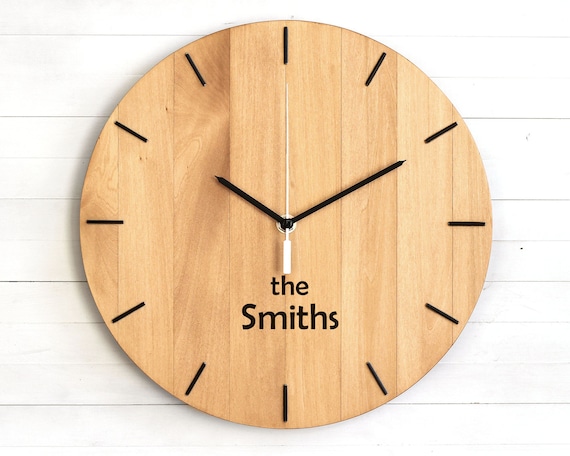The image showcases a round, wooden analog clock with a light brown, natural wood finish. The clock face is simple and minimalist, featuring black hash marks for each hour, without numerical indicators. The hour and minute hands are sleek, black metal, while the second hand is silver or white, pointing straight up, indicating that the time is exactly 10:10. Prominently displayed in black text on the clock face is the inscription "The Smiths," suggesting it may be a personalized item. The clock is mounted on a white wall adorned with horizontal light gray lines, resembling wooden planks and wood grain patterns, enhancing the rustic and elegant aesthetic of the scene.